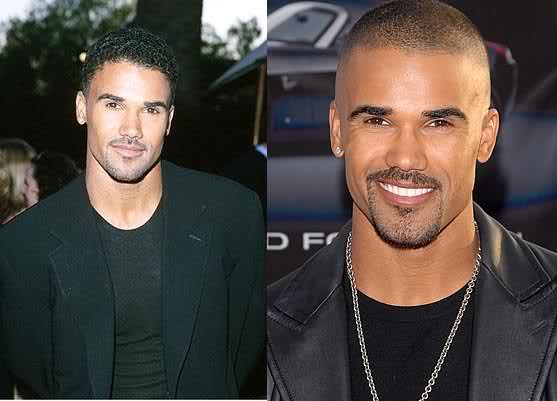The image showcases a contrast between two photographs of Shemar Moore taken at different times in his life, highlighting his evolving style. In the left photo, a younger Moore dons an open black suit jacket over a black t-shirt, revealing a modest amount of forehead hair and a thinner goatee. The backdrop includes blurry trees and people, adding a casual, outdoor ambiance. In the right photo, an older Moore appears, his hair cut significantly shorter with undercut sides, and sporting a thicker goatee. He wears a black leather jacket over a black shirt, accented by a white silver chain and a single stud earring on his left ear (right side of the photo). This image features a blurred sports car in the background, contributing to a more dynamic, urban atmosphere.